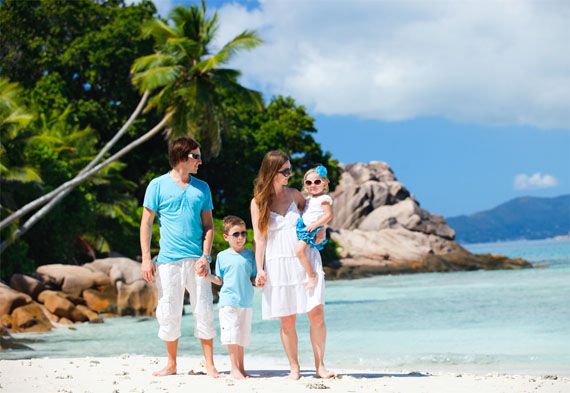The image captures a family enjoying a day at the beach, centered within a horizontally aligned rectangular frame. In the backdrop, a blue sky peppered with fluffy white clouds stretches overhead, while distant mountains or hills add depth to the scene. The right side showcases hints of the mountain range, while the left side is more lushly focused, featuring vibrant green leaves and a palm tree growing diagonally. 

The family, comprising a man, a woman, a young boy, and a toddler girl, stands barefoot on light tan sand right in front of the bluish-gray water, possibly part of a scenic bay or cove suggestive of a Polynesian island or Hawaii. Everyone sports sunglasses. The man, positioned on the left, wears a seafoam blue short-sleeve t-shirt and rolled-up white pants, glancing lovingly at his wife and kids. The young boy between the parents mirrors his father’s attire with a blue t-shirt and white shorts.

The woman in the middle is dressed in a flowing white sundress, her long brown hair cascading down as she cradles a little girl in her arms. The toddler, who also wears sunglasses, has a white short-sleeve top and a blue ruffled skirt, with a blue hair accessory. Both mother and daughter look towards the camera, adding a sense of connection to the viewer. Behind them, the palm tree's branch stretches across the image, complementing the serene and picturesque beach setting.